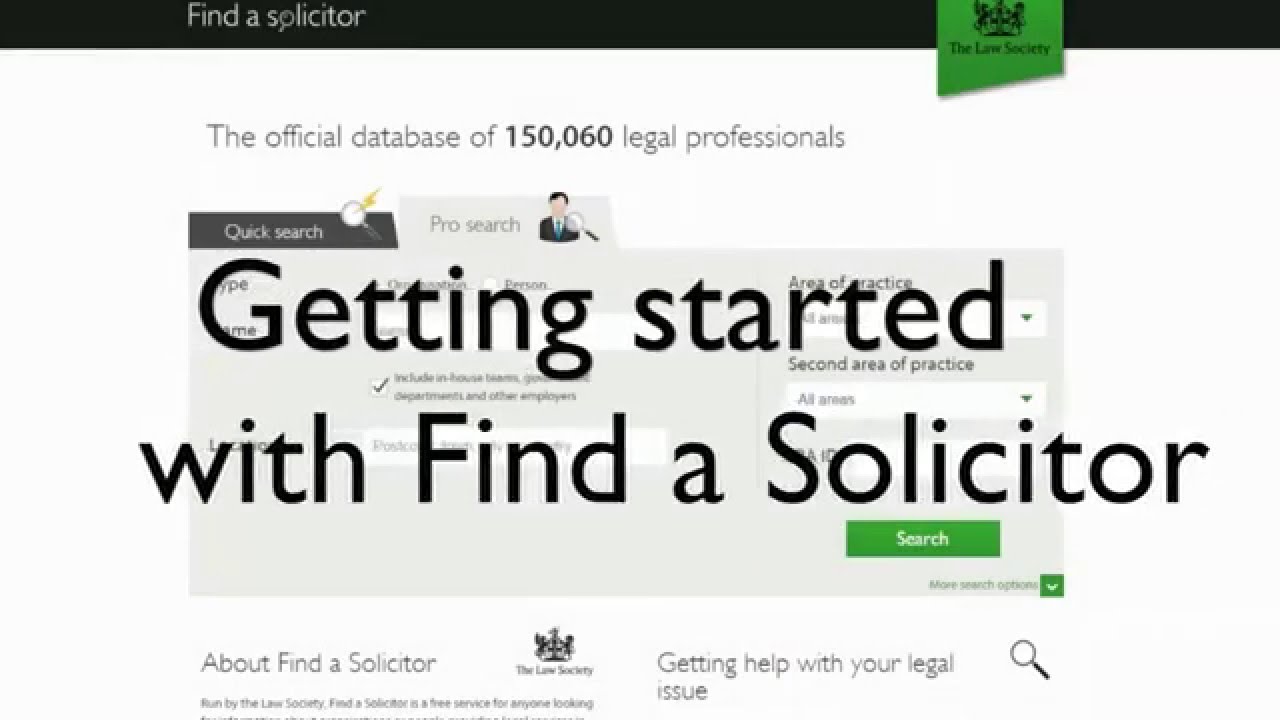The image shows a webpage with a detailed layout centered around finding a solicitor. At the very top, there is a narrow black horizontal banner stretching across the width of the screen. On the left side of this banner, there is a magnifying glass icon next to the text "Find a Solicitor." On the right side, there is a small green banner with the text "The Law Society."

Beneath this banner, a prominent text reads, "The official database of 150,060 legal professionals," with "150,060" in black and the rest of the text in gray. 

Further down, large black text says, "Getting started with Find a Solicitor," followed by a green search button. Below the button, there are two sections: "About Find a Solicitor" on the left bottom corner and "Getting help with your legal issue" on the right, both accompanied by a magnifying glass icon.

In the center of the screen, there is a light gray section displaying partial content under the message "Getting started with Find a Solicitor." It has two tabs labeled "Quick Search" and "Pro Search," with a light gray background and various search categories aligned to the right, providing a clear and functional layout for the users.